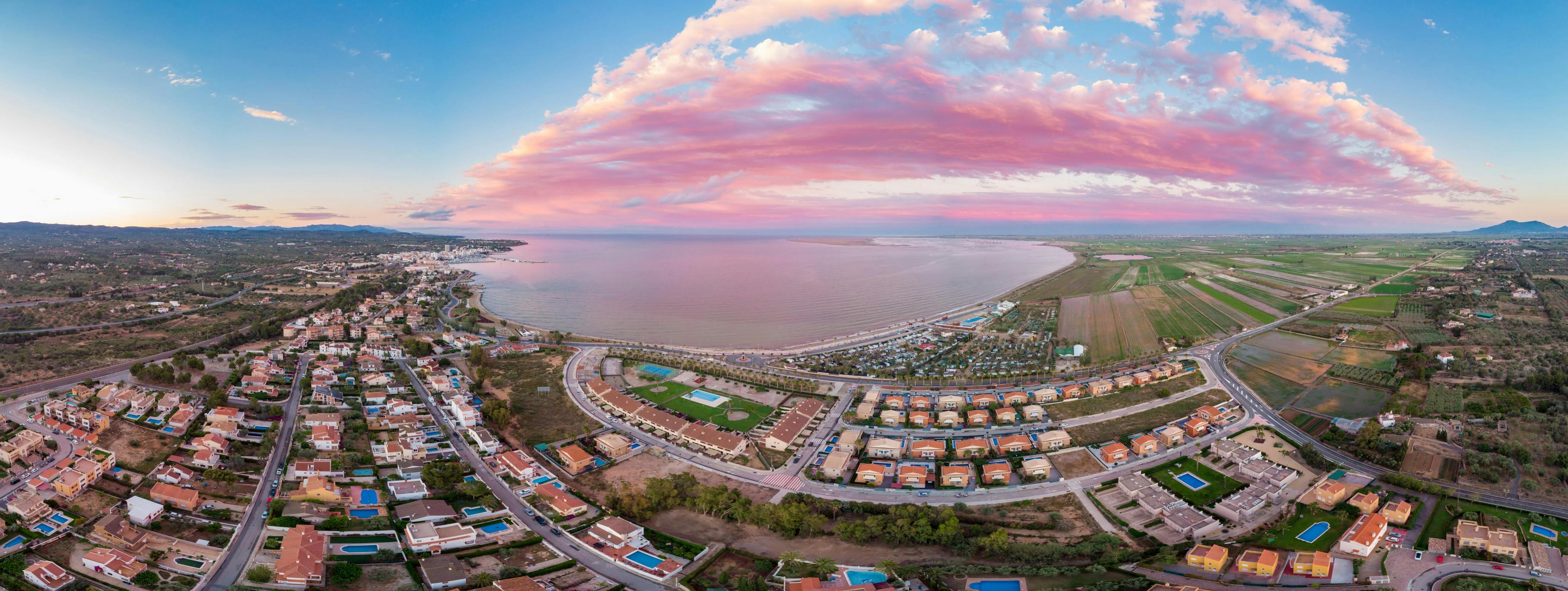This breathtaking panoramic photograph captures a vibrant cityscape under a mesmerizing sky. The image, which appears to have been taken with a fish-eye lens, features a large, still body of water at the center, reflecting the beautifully colored sky above. The sky transitions from blue on the outskirts to a vivid pink cluster in the middle, with clouds that have a distinct purple hue, adding depth and whimsy.

Surrounding the water, a sprawling network of streets and roads weaves through an array of residential houses, many of which sport red or reddish clay roofs. Scattered among these homes are notable landmarks, including what seems to be a sports field with distinguishable stands, perhaps for football, and various residential complexes with pools.

On the far left, the landscape transitions into a lush green area, possibly with dense foliage, while the far right reveals open tracts of land that look like farm fields. Distant mountain ranges create a picturesque backdrop on the far left of the image, adding a sense of grandeur to the scene. This aerial view beautifully highlights the juxtaposition of urban and natural elements, all under a sky painted with the hues of a setting sun.